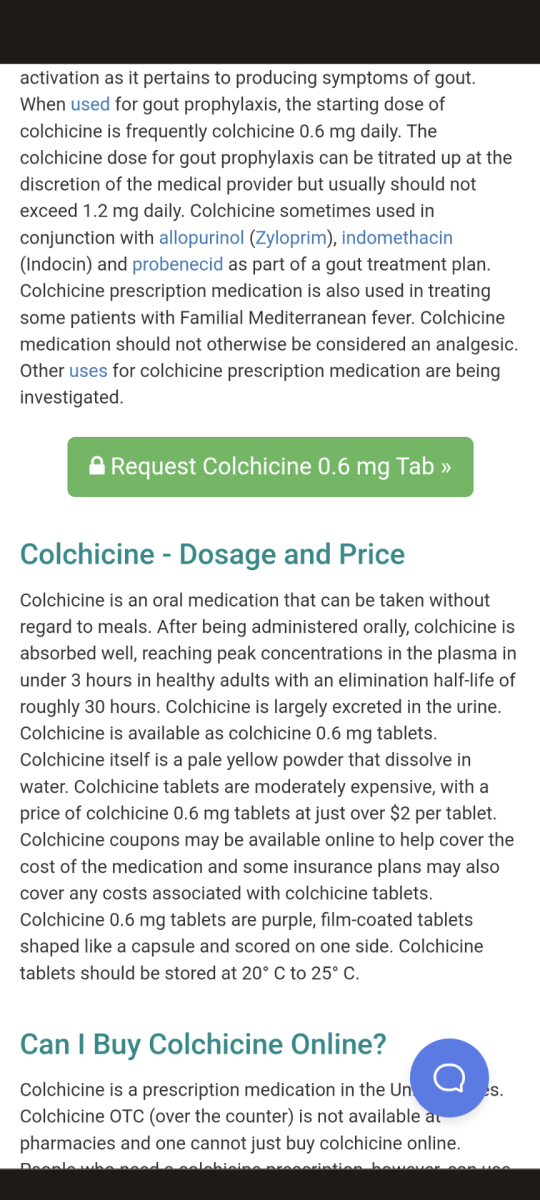A screenshot of a website delivers informative content about Colchicine, detailing its use and availability. At the top, a black navigation bar introduces the topic, focusing on gout symptoms. It emphasizes Colchicine’s common dosage for gout prophylaxis—0.6 milligrams daily—and mentions its potential use in combination with other medications, such as Allopurinol, Indomethacin, and Probenecid for gout treatment.

Central to the page is a prominent green button featuring a white lock icon on the left, labeled "Request Colchicine 0.6 mg tab," indicating a clickable option for more information or to request the medication. 

Further down, under a teal-colored header entitled "Colchicine Dosage and Price," the text describes Colchicine as an oral medication that can be taken regardless of meals. After oral administration, it is well-absorbed and reaches peak plasma concentrations within three hours in healthy adults.

Another teal header, "Can I Buy Colchicine Online," clarifies that Colchicine, being a prescription medication, is not available at standard pharmacies. Adjacent to this paragraph, on the right, is a circle icon with a chat bubble, likely offering a customer service chat option.

The webpage concludes with a black bar at the bottom, framing the detailed informational layout.